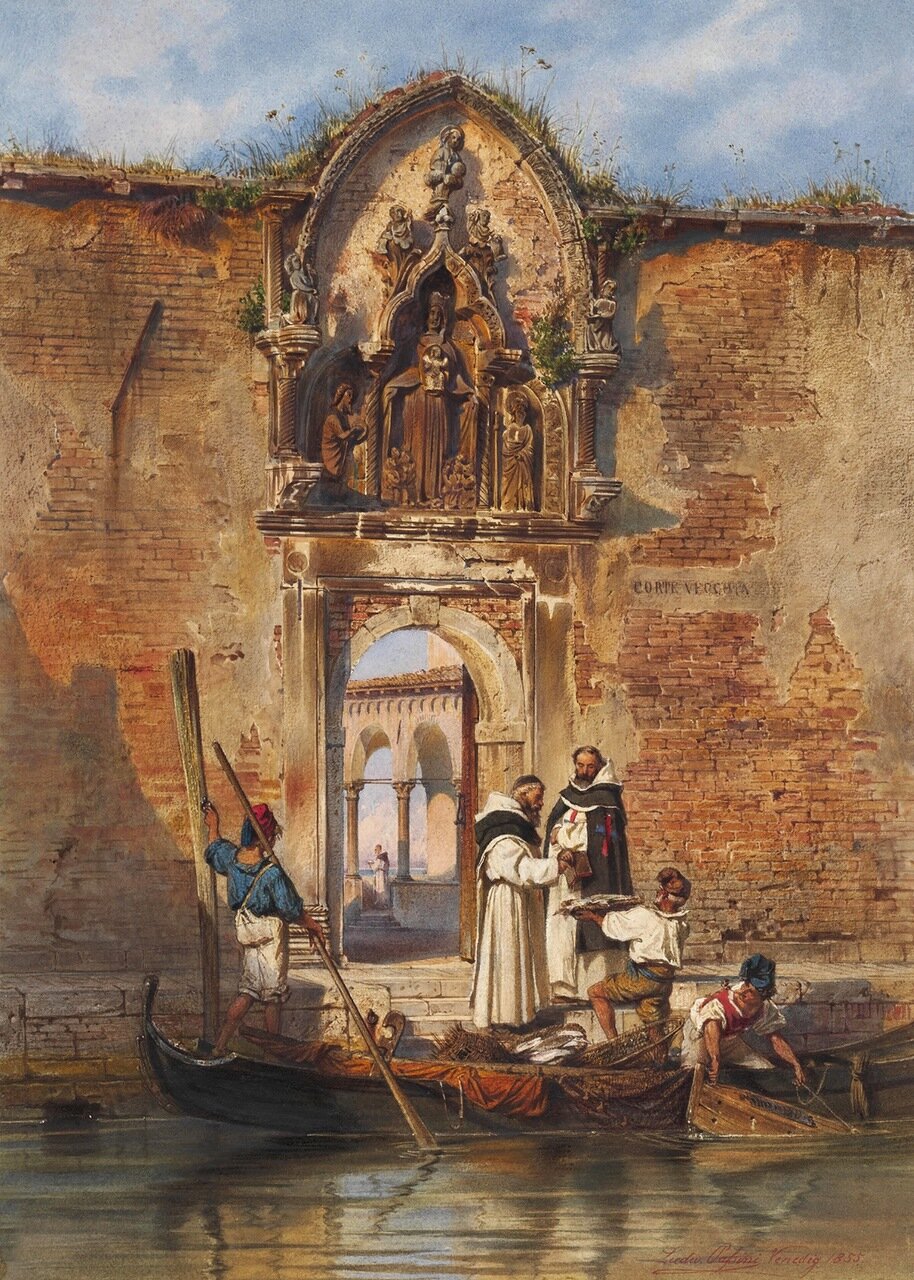In this detailed oil painting, a significant element is a grand, reddish-brown brick wall reminiscent of an ancient church or cathedral. Dominating the upper center of the wall is a beautifully carved inset, bordered by an arched dome, housing a religious scene. Central to this scene is a depiction of Jesus flanked by two figures praying on their knees. Surrounding Jesus are ornate columns and sculptures, possibly of angels, looking down protectively.

Below this religious tableau, an archway with an intricate frame leads into the structure, where a Venice-like canal unfurls in the foreground. Reflecting the grayish water, a gondola balanced delicately on the surface carries three individuals. One, a woman in a blue top, holds a large oar for steering, while a boy stands on the gondola offering a fish to two priests or holy men in white tunics with brown or gray capes. One of these priests is adorned with a cross marked by a vertical red and horizontal blue line.

The painting richly captures a blend of religious reverence and everyday activity, bridging the divine with the mundane in a scene evocative of historical depth and cultural interplay.